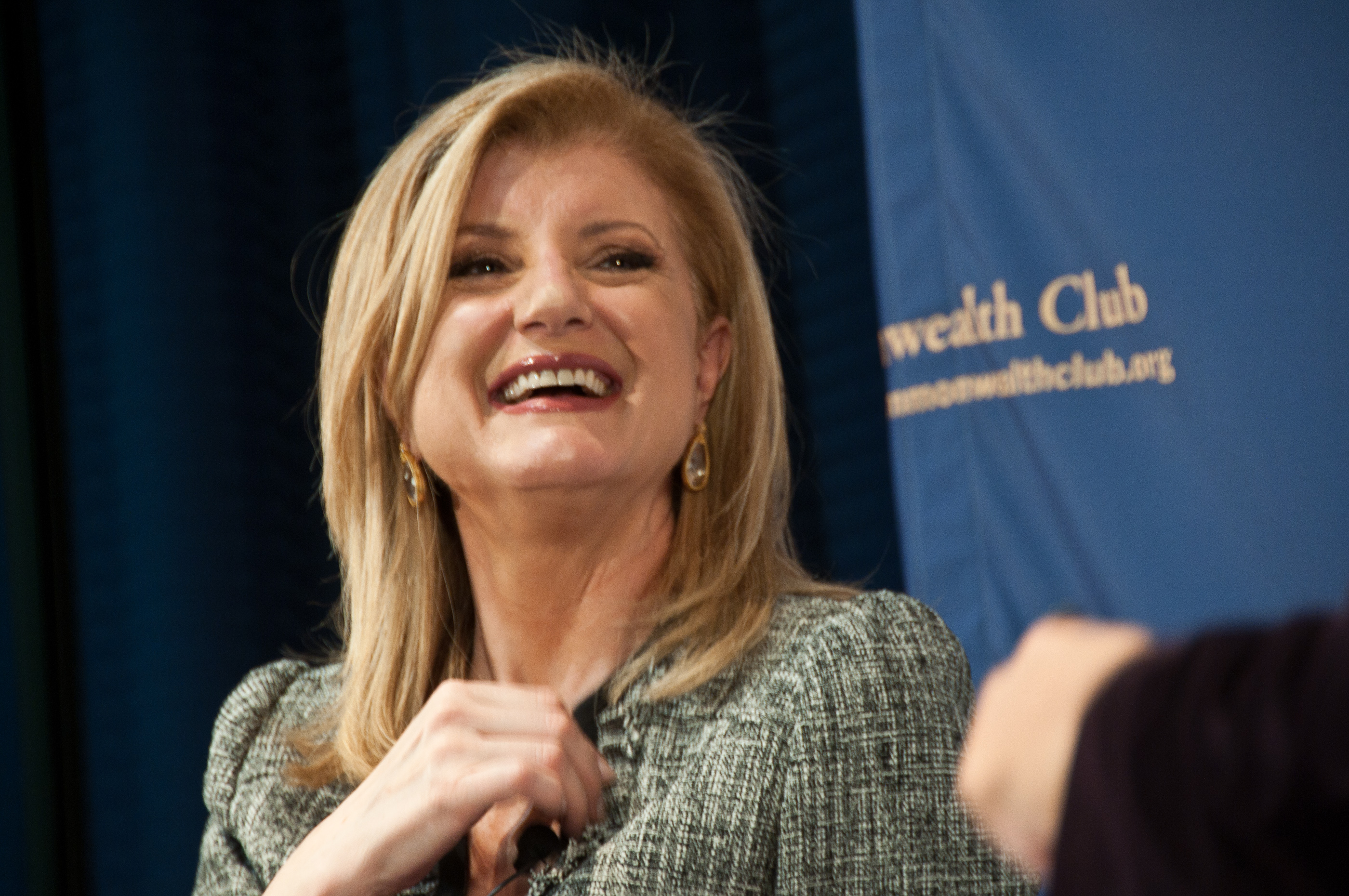This image captures a woman in her late 40s or early 50s with collarbone-length blonde hair, smiling broadly. She has dark eyes and is wearing reddish-dark pink lipstick. Her attire consists of teardrop-style gold earrings with a clear or purplish emblem in the middle, and a white and gray woven or tweed jacket over a black undershirt. The setting suggests she is seated, possibly on a stage or at an event, engaged in conversation with someone whose dark-clothed arm and hand are visible but blurry in the bottom right corner. Behind her, a dark blue curtain serves as a backdrop, displaying a banner with the partly obscured text: "Commonwealth Club," and a website, "commonwealthclub.org."